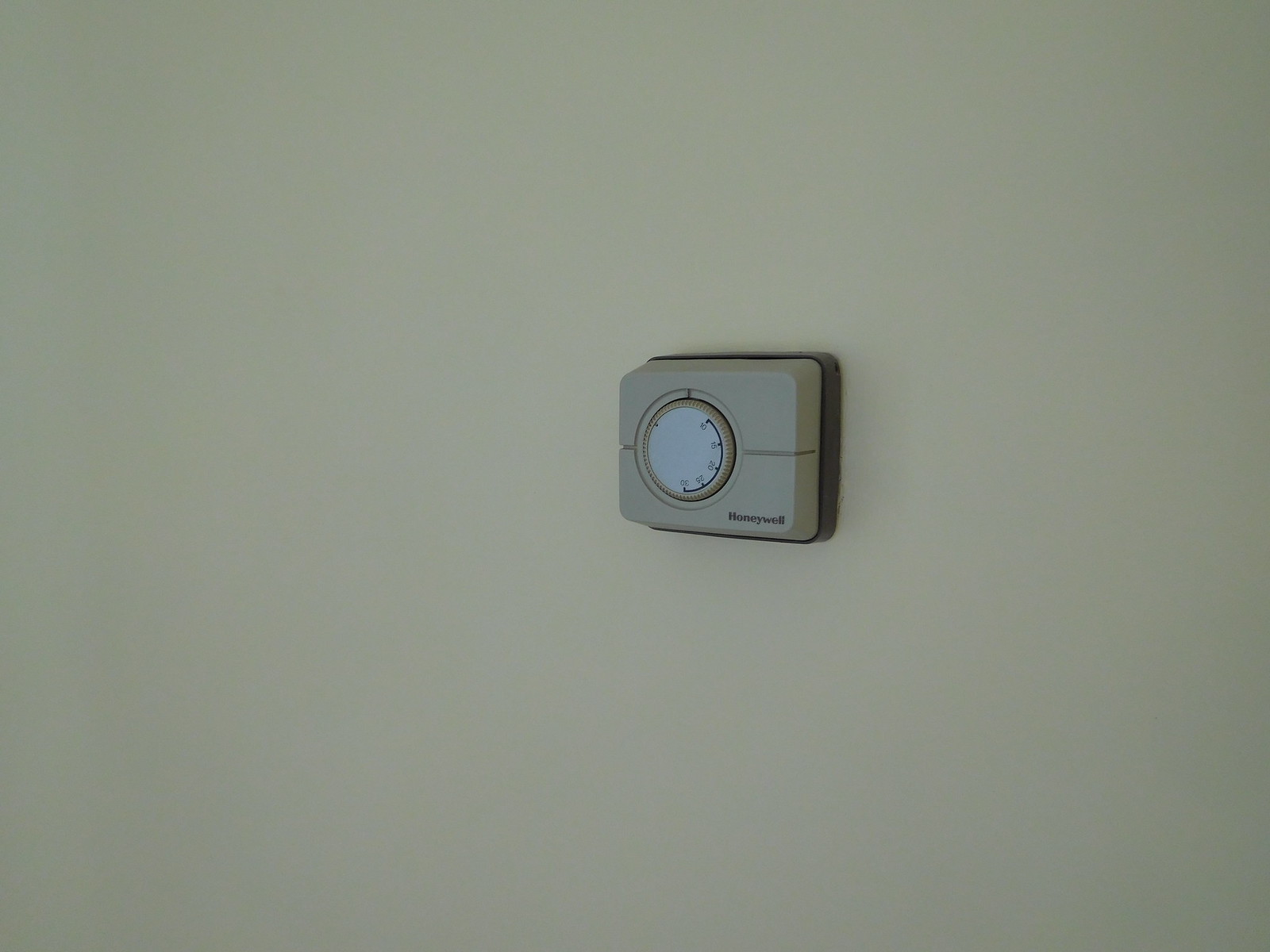The image depicts a vintage Honeywell thermostat mounted on a large gray wall. The device is a small, light gray metal box framed by a darker gray frame that secures it to the wall. Central to the thermostat is a prominent circular dial, encircled by numerous fine lines which likely serve as measurement markers. The outer edge of this dial features a series of numbers and a black indicator line, though the specific numerical values are somewhat difficult to decipher, raising questions about whether the scale is in Celsius or another unit of measurement. The iconic Honeywell name is printed on the lower right-hand side of the box, reinforcing the device's credibility. This analog thermostat is indicative of a time before digital advancements, and while it might traditionally be used to control temperature, its exact function here is uncertain, as Honeywell produces a range of electronic equipment including humidity controls. The overall aesthetic evokes a sense of nostalgic simplicity and precision engineering.